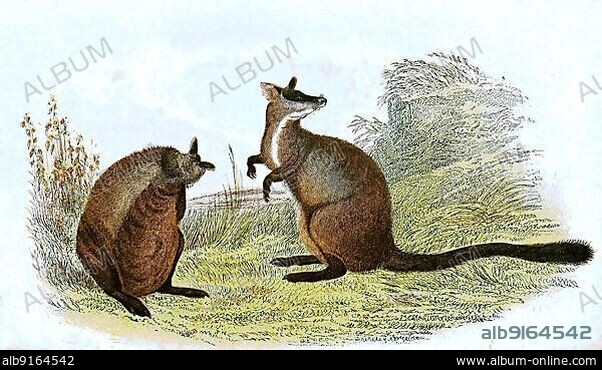This detailed image, bearing a watermark with multiple instances of "album" and text indicating "www.album-online.com" in the bottom right corner, depicts two unidentified mammals in a style reminiscent of Audubon's illustrations. Set against a faint, blue, wispy background indicative of cloud cover, these creatures stand in a green grass field. Both animals display kangaroo-like features with long feet and small upper arms; the one on the left is stout, dark brown, and appears to be grooming its back with visible perky ears. It lacks a distinct tail. The animal on the right, slightly taller with a long, bushy-ended tail, has its body facing left while it gazes backward over its left shoulder. Their anatomy is a mix, possessing cat-like front paws and rabbit-like bottom feet, creating an intriguing and somewhat ambiguous portrayal. The bottom corners of the image also display the code "ALB9164542".